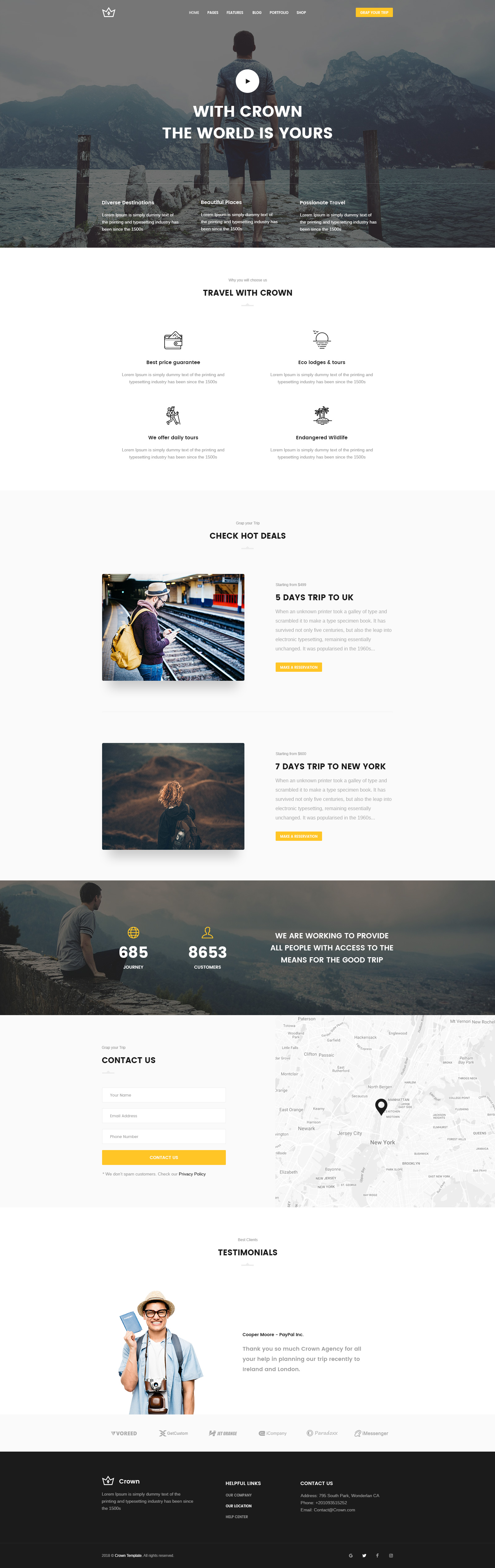This image depicts a sleek, modern travel website with a long, narrow layout, approximately three to four times as tall as it is wide. The website features high-quality, artistic photographs, enhancing its visual appeal.

At the very top of the page is a panoramic banner image of a man standing on a dock, gazing at towering mountains shrouded in voluminous clouds. This banner includes an opaque orange rectangle in the upper right corner with illegible white text and a white play button, indicating a video.

Beneath the banner, a prominent tagline reads, "With Crown, The World is Yours," accompanied by several unidentified white boxes. Following this section is a large white box with the text "Travel with Crown" and four small icons with descriptions, which are not clearly legible.

The next section features a grayish box promoting travel deals. One photo shows a man at an airport, advertising a "Five Days Trip to the UK," while another image depicts a person on a mountain range, promoting a "Seven Days Trip to New York." Below, there's an image of a man sitting on a ledge, overlooking a scenic mountain view.

Towards the bottom of the website is a map image accompanied by a "Contact Us" form on the left, providing white input boxes for user information and an orange "Send" button. Finally, a "Testimonials" header introduces a quirky-looking man wearing a safari hat and holding a passport, smiling at the camera.